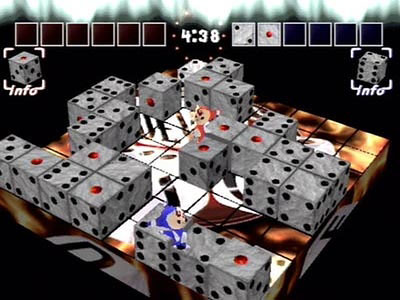The image depicts an intricate arrangement of dice, meticulously stacked to form a mini-game tableau for several characters. At the top center, a timer displays the number "438," indicating a countdown. Flanking the timer, there are two white squares designated for holding dice: the square on the right contains a die showing the number "2" and another showing "1," while the square on the left remains empty. In the top-left corner, a die with the label "info" is prominently visible, mirrored by an identical die in the top-right corner. Two animated characters, one blue and the other red, appear to be enthusiastically breakdancing within the scene, adding a dynamic and playful element to the setting.